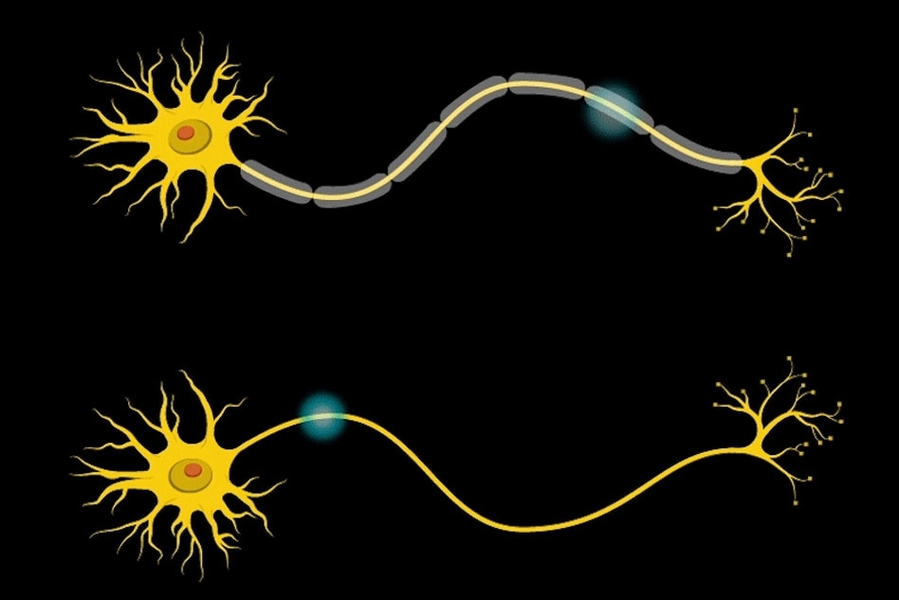The image is a horizontal, rectangular picture with a black background, potentially representing microscopic nerve cells or optic nerves. Dominating the image are two nearly identical structures, resembling nerve cells with rounded centers that classically depict a nucleus. These parts are yellow and have branching projections akin to dendrites, capturing the nerve-like feel. The cells' centers look somewhat like olives with a pimento in the middle. From each cell, a curvy, glowing line extends rightward, reminiscent of an axon trailing off from a nerve cell body. The upper line has a lighter yellow hue with a radiant glow, whereas the lower line is a solid yellow. Both lines culminate in more branching, dendrite-like endings. This vividly detailed image lacks any textual descriptions or labels.